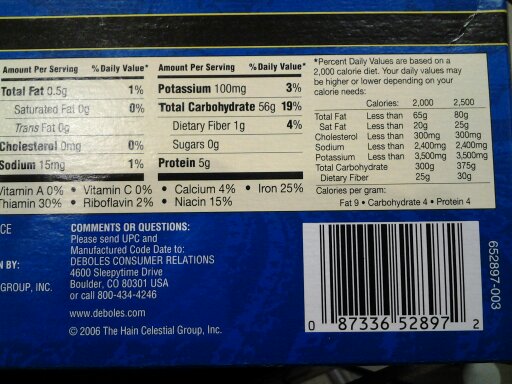This photograph captures the back of a food package featuring detailed nutritional information against a striking navy blue background. The bottom right corner prominently displays a UPC code: 087336528972, in the classic black-and-white striped format. At the top of the packaging, a black and yellow strip adds a visual highlight, extending horizontally across.

The nutritional facts are presented in a clear, white box with black text. The breakdown begins with the amount per serving, noting total fat content at 0.5 grams, saturated fat at 0 grams, trans fat at 0 grams, and cholesterol at 0 milligrams. Sodium content is marked at 15 milligrams. The daily value percentages are specified as follows: Total Fat 1%, Saturated Fat 0%, Trans Fat 0%, Cholesterol 0%, and Sodium 1%.

Further details highlight vitamin and mineral content: Vitamin A at 0%, Thiamine at 30%, Vitamin C at 0%, Riboflavin at 2%, Calcium at 4%, Niacin at 15%, and Iron at 25%. Additionally, the potassium content is 100 milligrams (3% daily value), carbohydrates are listed at 56 grams (19% daily value), dietary fiber at 1 gram (4% daily value), with 0 grams of sugars, and 5 grams of protein.

At the bottom of the nutritional information, a note is included for customer feedback: "Comments and questions, please send UPC and manufacturer code date to Debole's Customer Relations, 4600 Sleepy Time Drive, Boulder, Colorado, 80301 USA."